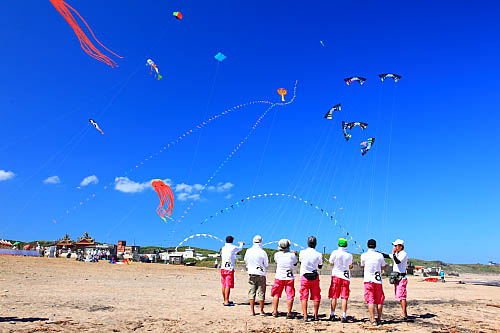This vibrant, overexposed photograph captures a lively scene at a beach on a bright, sunny afternoon with an intensely dark blue sky fading to a paler shade at the horizon. Dotted across the sky are twelve colorful kites in various shapes, including black and white manta ray-shaped kites with bright stripes, large orange and red jellyfish-like kites, a blue diamond-shaped kite, a green and red kite, and a giant multicolored fish kite. Fluffy clouds are sparsely scattered in the upper left corner of the image.

In the middle foreground, seven men stand with their backs to the camera, all dressed in white polo shirts bearing the number eight and mostly sporting pink shorts, with the exception of one man in dark green shorts. They wear assorted caps: bareheaded, white hat, white hat, brown or gray hat, green hat, bareheaded, and white hat. Each man is flying or appears to be flying similar-looking black-and-white kites, which add to the spectacle in the sky. Occasionally, it seems some individuals may be controlling multiple kites, given the visible tangle of strings.

The sandy beach transitions into green rolling hills in the distance, where small booths and tents suggest a bustling gathering or a camping site, and possibly even a small restaurant. This scene captures the playful and colorful essence of a beach outing, with the sky filled with an eclectic mix of kites soaring high.